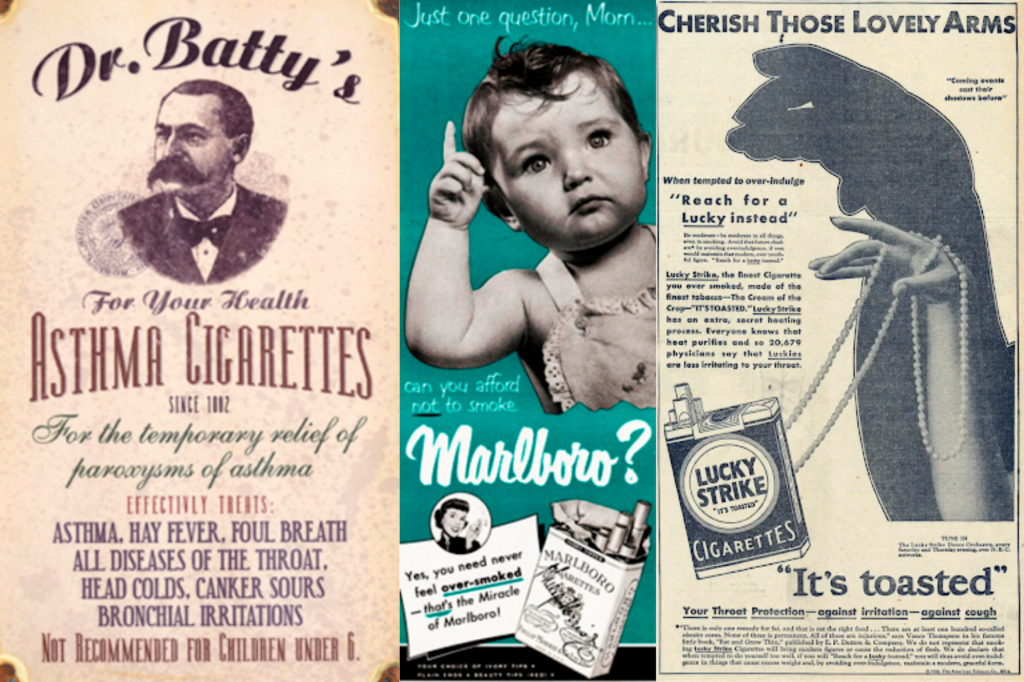The image displays three vintage cigarette advertisements, showcasing the marketing tactics from different eras. 

The first ad is for Dr. Batty's Asthma Cigarettes, dating back to 1882. It promotes the cigarettes as a remedy for a variety of ailments including asthma, hay fever, foul breath, throat diseases, head colds, and canker sores. The advertisement features a man with a big mustache, dark hair, a bow tie, and a suit, and cautions not to use the product for children under six.

The second ad, likely from the 1940s, is for Marlboro cigarettes. It features a baby in overalls raising a finger, accompanied by the text, "Just one question, mom. Can you afford not to smoke Marlboros?" This ad emphasizes the supposed mildness and the idea that "you need never feel over-smoked," and includes an image of a Marlboro cigarette pack.

The third ad is for Lucky Strike cigarettes, with the slogan "Cherish those lovely arms. Reach for a Lucky instead." The phrase "It's toasted" is highlighted at the bottom. This advertisement showcases a hand holding a cigarette with a pearl necklace in the background, adding an air of elegance to the product. These ads together provide a fascinating glimpse into early 20th-century cigarette advertising.